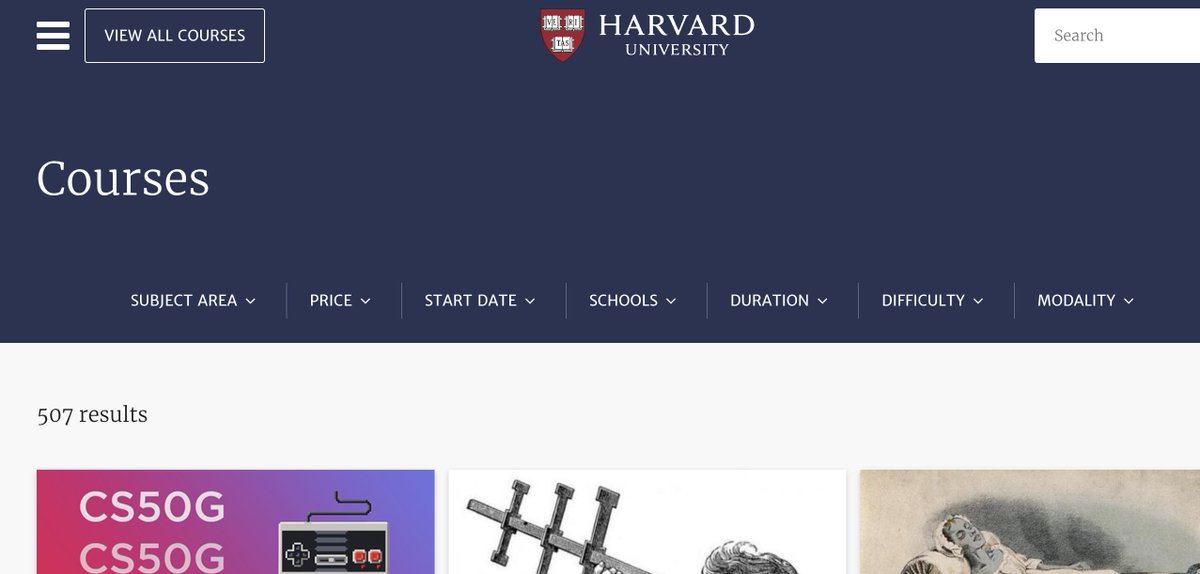The image is a screenshot of a website, prominently featuring a large dark navy blue banner across the top. In the top left corner, there are three horizontal lines in white, indicating a menu. Adjacent to this, outlined with a thin white line, is white text in capital letters that reads "VIEW ALL COURSES." On the far right side of the banner is a search bar, which is white and contains the word "SEARCH" in blue.

Centrally positioned in the banner is a coat of arms shield displaying three open books against a red background, accompanied by the text "Harvard University" beneath the shield. Below this, on the left side of the banner, is the word "COURSES" in large font. Across the bottom of the blue banner are several dropdown options labeled: "Subject Area," "Price," "Start Date," "Schools," "Duration," "Difficulty," and "Modality."

Below the dark blue banner, the website screen transitions to a white background. In the top left corner of this white space, it shows a count of "507 results." Immediately visible are three course thumbnails. The leftmost thumbnail features a gradient background transitioning from dark pink to lilac mauve, with white text that reads "CS50G" twice, accompanied by an image of a game controller. The central thumbnail has a white background with an indistinct gray drawing. The third thumbnail on the right has a vintage aesthetic, depicting a woman in a bonnet lying on a bed.